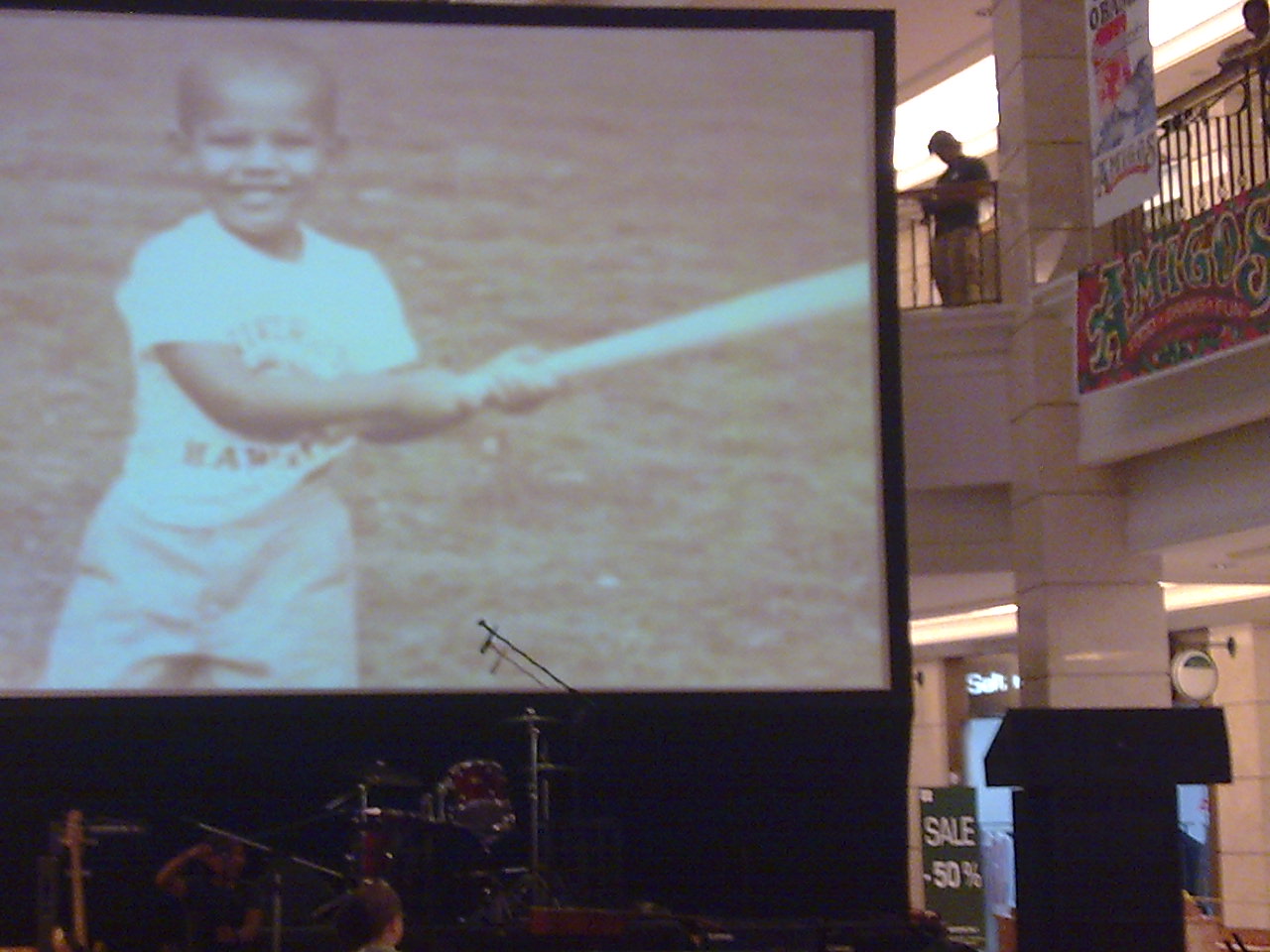The image captures a large indoor atrium, potentially set in a mall, featuring a prominent stage area. Dominating the background is an immense projector screen with a black outline, displaying a photograph of a smiling, dark-skinned toddler. The child, dressed in a white short-sleeved t-shirt and white shorts, holds a white baseball bat mid-swing, against a grassy backdrop. In front of this screen, a full drum set is arranged, with a microphone stand positioned in such a way that the microphone intersects the bottom edge of the screen. To the right of the stage, at the bottom of the photo, stands a dark-colored podium. Adjacent to this setup, the upper right corner reveals a second-floor balcony with beige block columns, where a dark-shirted gentleman in tan pants and another unidentified individual stand, leaning on the railing as they observe the scene below. Additionally, there is mention of retail signs such as a "sale 50% off" and a "banner for amigos," hinting at a commercial setting prepared for an event.